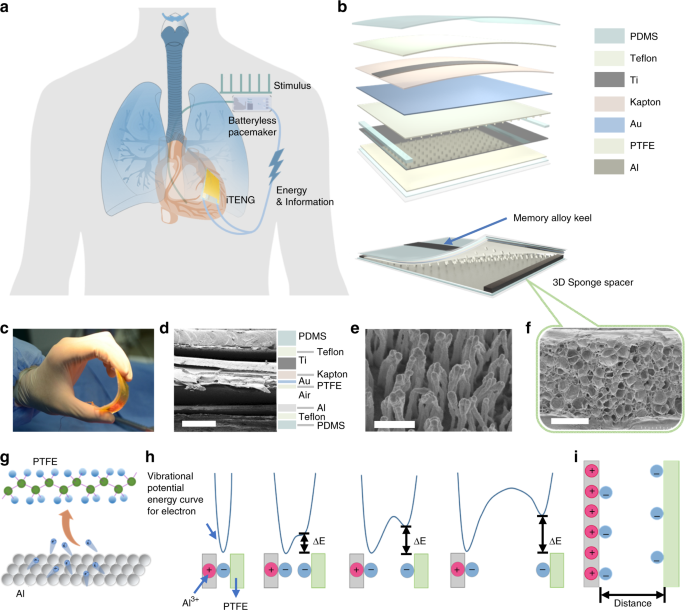The infographic set against a solid white background illustrates the detailed anatomy and functionality of a battery-less pacemaker within a human body. At the center is an outline of a person's torso highlighting the lungs and the pacemaker. Below and to the right, various diagrams and images are segmented by letters A through I. Square A at the top reveals the lungs and a battery-less pacemaker, overlaid with color-coded layers and blocks detailing different functional modalities.

Square B focuses on the layered structure of the device, supported by a color-coded key. Square C depicts a surgeon holding the pacemaker part. Squares D, E, and F showcase microscopic images of the device's layers in black and white. Squares G, H, and I offer detailed diagrams of the atoms and molecules involved. Additionally, there is a mapping of energy, information flow, and vibrational potentials represented by colored markers, arrows, and layers throughout the infographic.